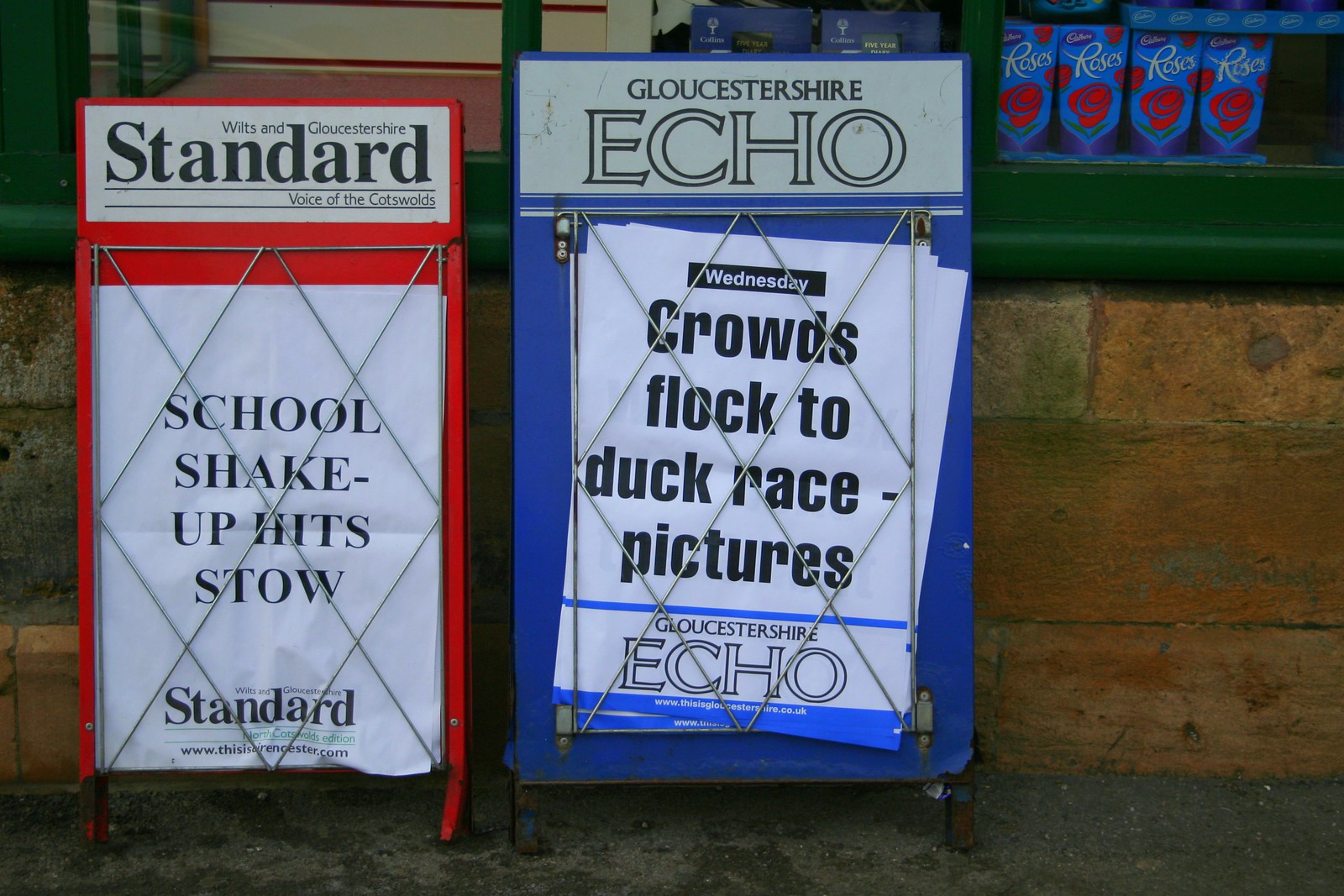This photograph captures two newspaper stands outside a small storefront. The stand on the left is red and labeled "Waltz and Glostschirr Standard, a voice of the Cotswolds" at the top, with a white paper featuring the headline "School Shake-Up Hits Stow." The right-hand stand is blue, labeled "Glostschirr Echo," showcasing a paper that reads "Crowds Flock to Duck Race Pictures" in black font. Both stands sit on dark green pavement, and the background reveals a brown brick wall with a green-bordered window displaying various products. The overcast or rainy ambiance adds a somber tone to the scene.